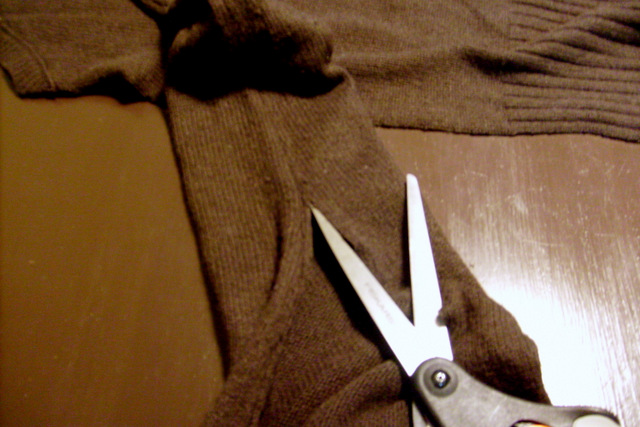In this image, a rich brown wooden table is prominently featured, subtly illuminated by an overhead light that creates a gentle glare, making the table’s color appear deeper and more pronounced on the left side. Centrally positioned on the table is a brown wool sweater, with its surface slightly textured and ribbed, particularly noticeable in the sleeve area on the top right, indicating where the wrist and forearm would be. On top of the sweater rests a pair of silver-metal scissors, their grayish handles connected by a small pin that attaches the sharp metal blades. The scissors are open, with the blades positioned in front of the sleeve, creating a striking contrast against the soft fabric of the sweater.